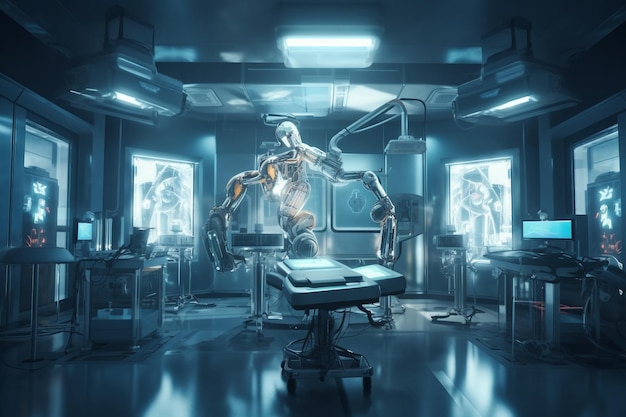This hyper-realistic computer-generated image depicts a futuristic medical laboratory bathed in a blue and silver color scheme, resembling a scene from a sci-fi movie. At the center of the room stands a metallic humanoid robot, characterized by its narrow torso and long, non-human arms, suggesting it's a sophisticated medical or surgical device. In front of the robot lies an operating table, indicative of its likely medical function. The high-tech room is illuminated by bright, space-age lighting both from the ceiling and walls, with various electronic panels and monitors contributing to the high-tech ambiance. The shiny, dark blue floor and several tables holding sleek, horizontal screens and various pieces of advanced machinery further emphasize the laboratory's futuristic and technologically advanced nature. The entire scene is filtered in shades of blue, with the robot and lighting fixtures rendered in silver and white.